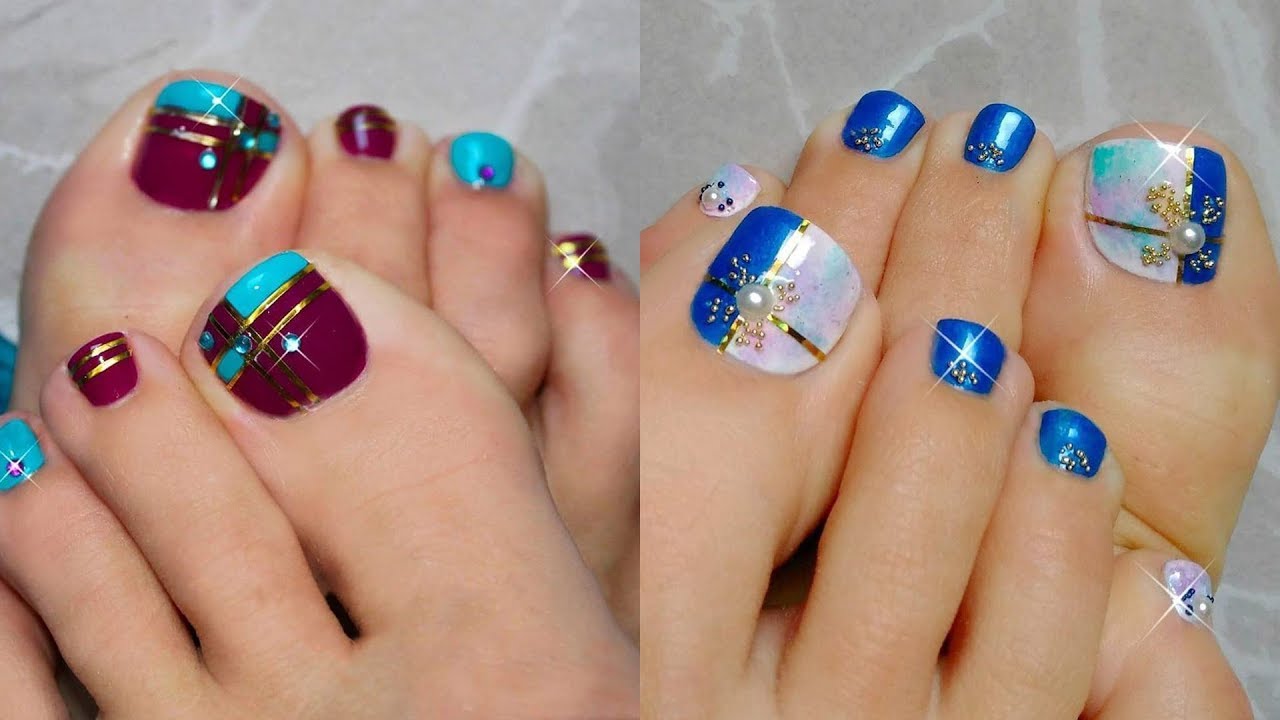This is a horizontally aligned rectangular image, where two square photographs are placed side by side with a slight overlap. Both photographs feature ornately decorated toenails set against a marbled gray and light gray background. The left side displays a right foot slightly angled beneath a left foot. The big toes boast a dark red polish adorned with gold stripes, glittering blue dots resembling stars, and rectangular sections of blue with tiny blue beads. The second toes have dark red polish with gold accents, while the third toes are primarily blue with a purple gem. The right side differs in color scheme and arrangement, showcasing a left foot placed on top of a right foot. The big toes here feature a marbled pattern of purple, green, and white with a vertical strip of bright blue, tiny pearls, and gold decorations. The second and third toes are predominantly solid bright blue with slight gold embellishments. The nails across both sets of feet are so meticulously decorated they appear almost like decals or fake nails, fitting perfectly over the natural nails.